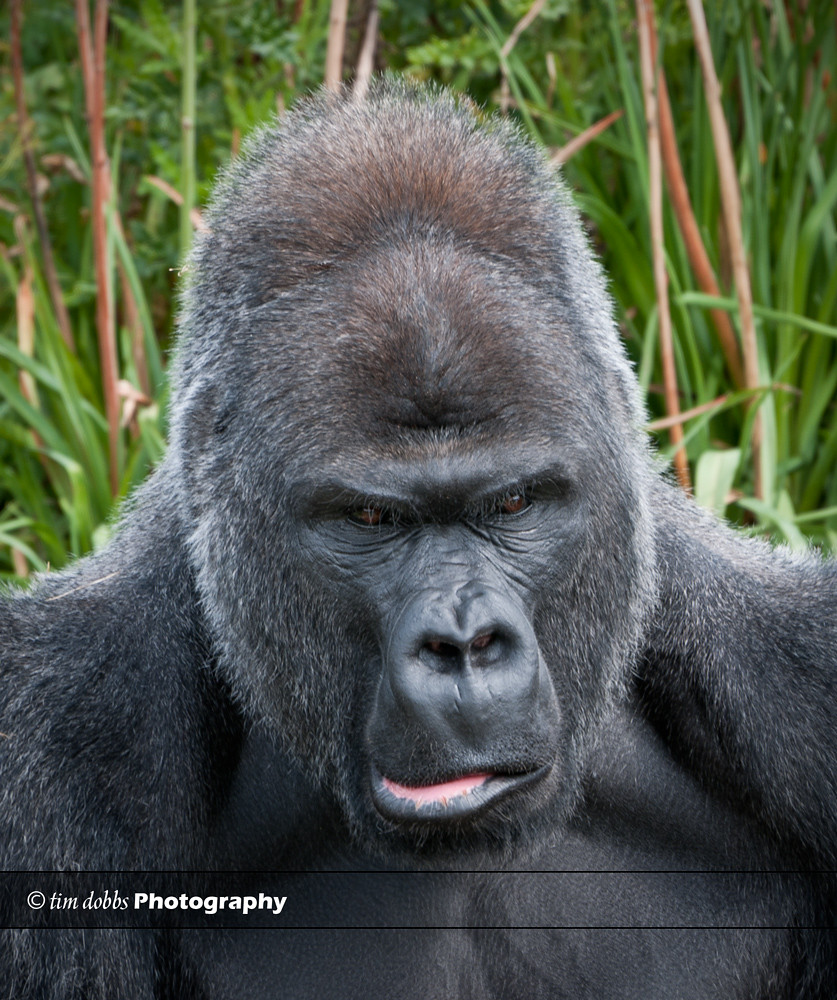The image is a close-up photograph of a large, powerful black gorilla, captured by Tim Dobbs Photography. The gorilla, likely a male, has a distinctive silver sheen to his black hair and a patch of reddish-brown hair atop his head. His stern, serious eyes are brown, and his bottom lip is slightly puckered open, revealing a pink tongue. He appears to be sitting in a lush outdoor setting with green grasses, reeds, and large brown branches behind him. The background is filled with greenery, including tall bamboo or reedy grass and bushes. In the bottom left-hand corner, a small black banner reads "© Tim Dobbs Photography."